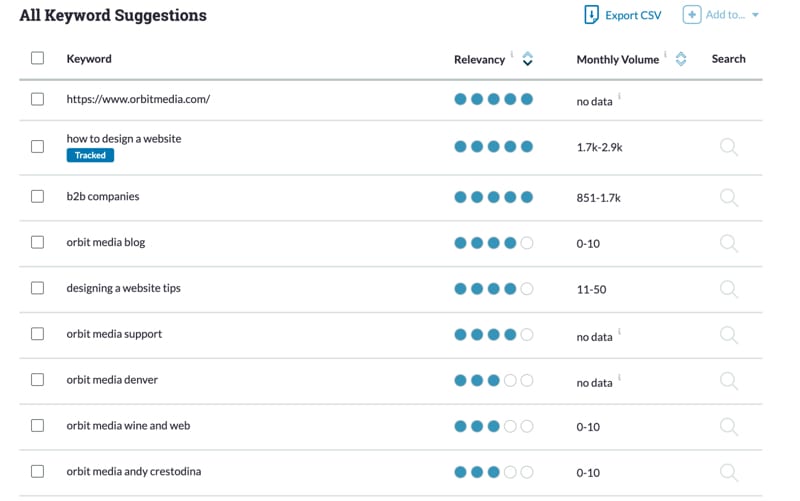Here is a cleaned-up and detailed caption for the described image:

---

The image displays a webpage from Orbitmedia.com that lists all keyword suggestions in a structured table format. The table consists of several columns titled "Keyword Relevancy," "Monthly Volume," and "Search." The contents of the table include various entries such as "How to Design a Website," "B2B Companies," "Orbit Media Blog," "Designing a Website Tips," "Orbit Media Support," "Orbit Media Denver," "Orbit Media Wine and Web," and "Orbit Media Andy Crestodina."

The top three entries are highlighted as the most relevant. The "How to Design a Website" keyword has the highest monthly volume, with views ranging between 1,700 and 2,900. Each row in the table features a "Search" button, which likely provides external links for further information. Additionally, there is an "Export CSV" button located at the top of the page, enabling users to download the data in a comma-separated values format, suitable for Excel spreadsheets.

The page has a clean, white background with primarily black text, while the relevancy ratings are accentuated in blue.